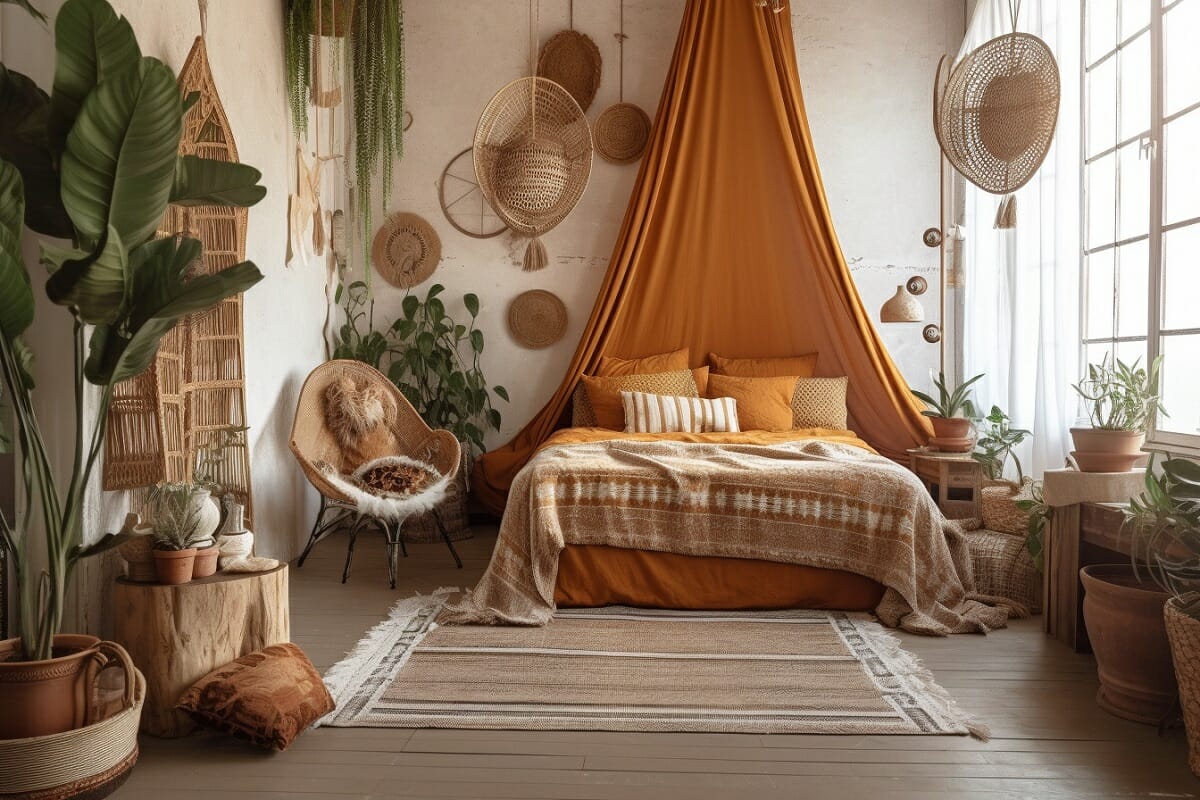This image captures a bohemian-styled bedroom bathed in soft, filtered light from a large window on one side of the room. The focal point is a queen-sized bed centered against the far wall, adorned with a rich blend of orange, brown, and beige pillows and a Native American-inspired bedspread. A large, billowing orange-brown drape descends from the ceiling, adding a dramatic touch behind the bed. The room exudes an earthy and organic vibe with its white walls and brown wood-paneled floor. Natural elements dominate the décor, including numerous potted plants scattered throughout, hanging plants above, and a large green palm positioned near the bed. Wicker elements are prevalent, with numerous woven baskets decorating the space and a wicker chair draped with a white fur blanket placed to one side of the bed. Additional touches include a beige rug with white tufts, a small table fashioned from a tree stump, and several smaller planters with cacti and other plants, enhancing the room’s natural aesthetic.